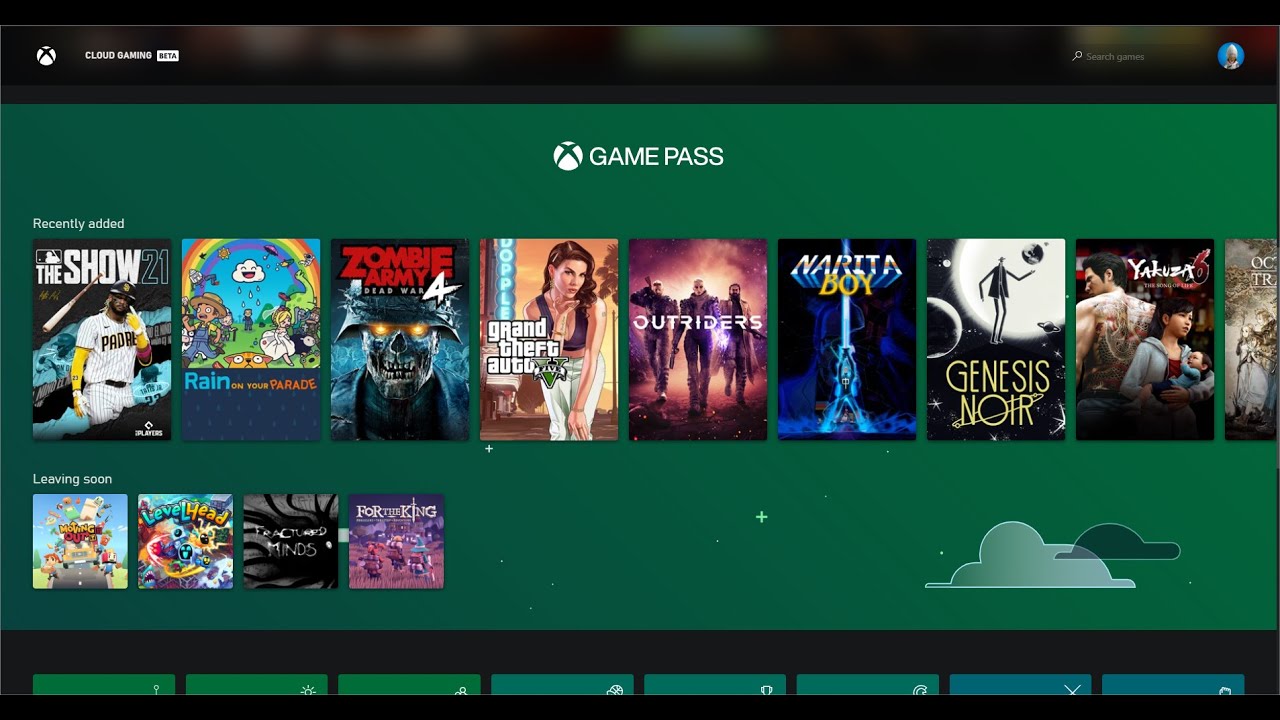This image, sourced from a website, prominently features the text "Game Pass" against a vibrant green background. In the upper-left corner, there is an icon, likely representing cloud gaming, depicted as a white circle with black breaks. Opposite to this, on the right side, there's an icon resembling a search bar set against a blue background, which includes a small, indiscernible cartoon character.

Below the "Game Pass" header, the section titled "Recently Added" showcases several game titles. These include:
- "MLB The Show" with an accompanying image of a baseball player
- "Rain On Your Parade," featuring an image of a rainbow and cartoon characters
- "Zombie Army 4" 
- "Grand Theft Auto V" with an illustration of a woman bending down
- "Outriders," displaying characters against a fiery backdrop
- "Narita Boy"
- "Genesis Noir"
- "Yakuza," with the title partially cut off 

The next section, labeled "Leaving Soon," presents four game thumbnails featuring various cartoon characters, albeit at a smaller scale.

Over to the right side of the image, there is a light green cloud icon paired with a darker green cloud. Below this, there are additional boxes aligned horizontally, although they are cut off and their contents are not visible. 

Overall, the image likely serves as a promotional banner for the Xbox Game Pass, highlighting the latest additions and upcoming departures in their gaming library.